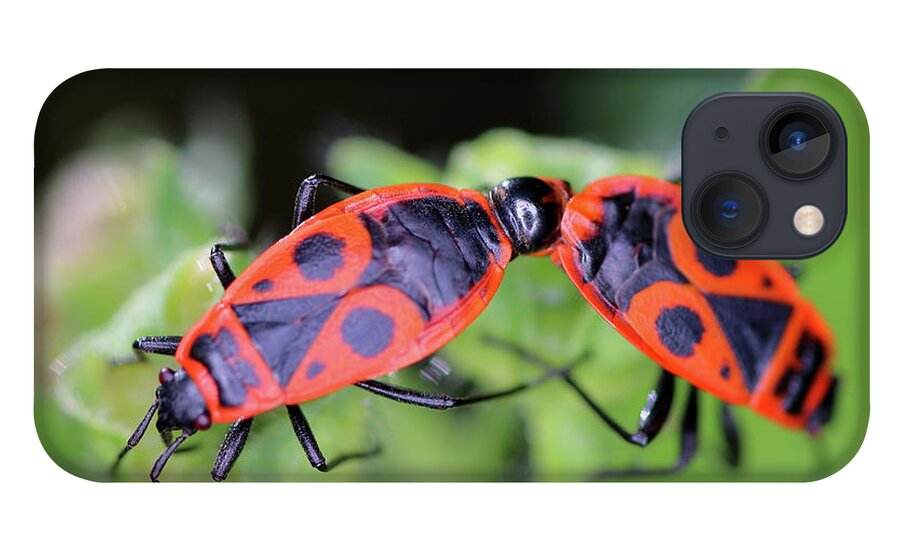The image depicts a detailed close-up of a high-tech phone case, likely for an iPhone, featuring an arresting design of two red and black insects. The insects are central in the composition, set against a blurred, leafy green background that subtly hints at foliage, enhancing the focus on the creatures. The insects themselves are elongated with vibrant red thoraxes adorned with an intricate pattern of black geometric shapes, including triangles and circles. Their segmented bodies and distinct features such as red eyes and multiple legs are meticulously rendered. In addition to the striking insect design, the phone case prominently shows the Apple iPhone's camera setup, including two camera lenses and a focus light, indicating the modernity of the device it encases. The case captures a vivid contrast between the sharp, detailed insects and the softly out-of-focus greenery, creating a unique and visually compelling accessory for the smartphone.